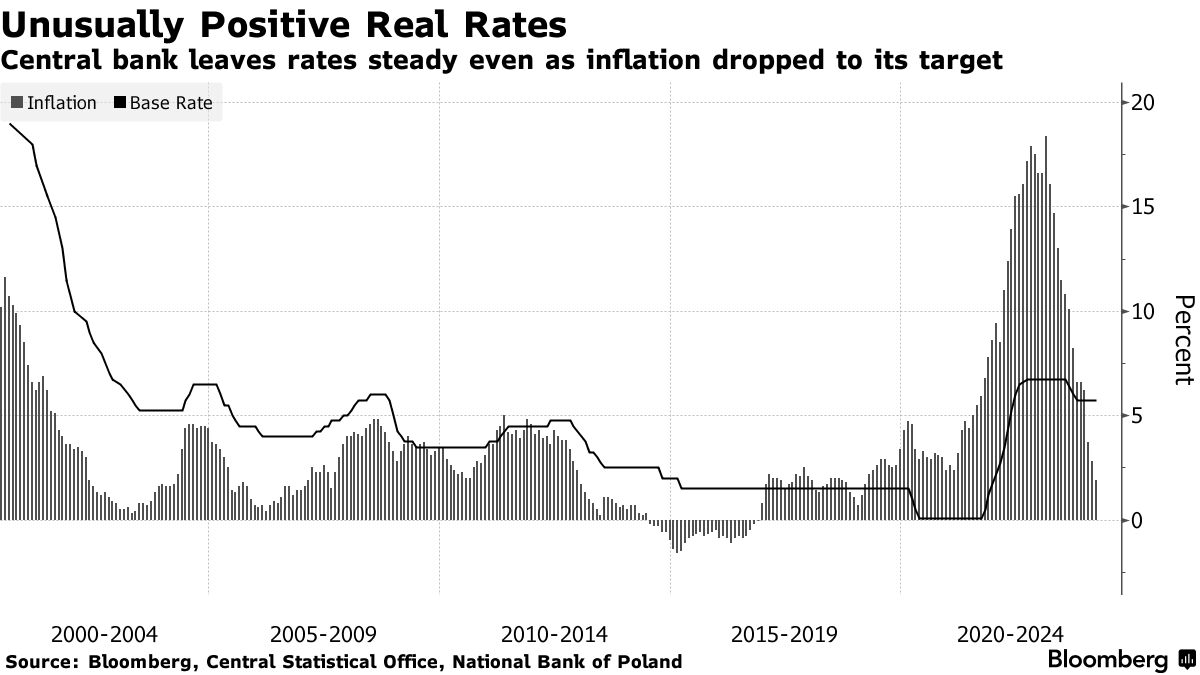The image is a detailed black and white chart with the title "Unusually Positive Real Rates, Central Bank Leaves Rates Steady Even as Inflation Drops to its Target," sourced from Bloomberg, the Central Statistical Office, and the National Bank of Poland. The chart expertly illustrates trends in inflation and the base rate from 2000 to 2024, with data presented in 5-year increments: 2000-2004, 2005-2009, 2010-2014, 2015-2019, and 2020-2024. A key on the chart distinguishes between inflation, shown as a lighter shaded bar graph, and the base rate, depicted as a darker line graph that fluctuates over the years. The vertical axis on the right side measures percentages from 0 to 20, highlighting the variations in economic indicators over the specified period. The chart efficiently communicates statistical trends with clarity and precision, serving as a reliable informational resource.